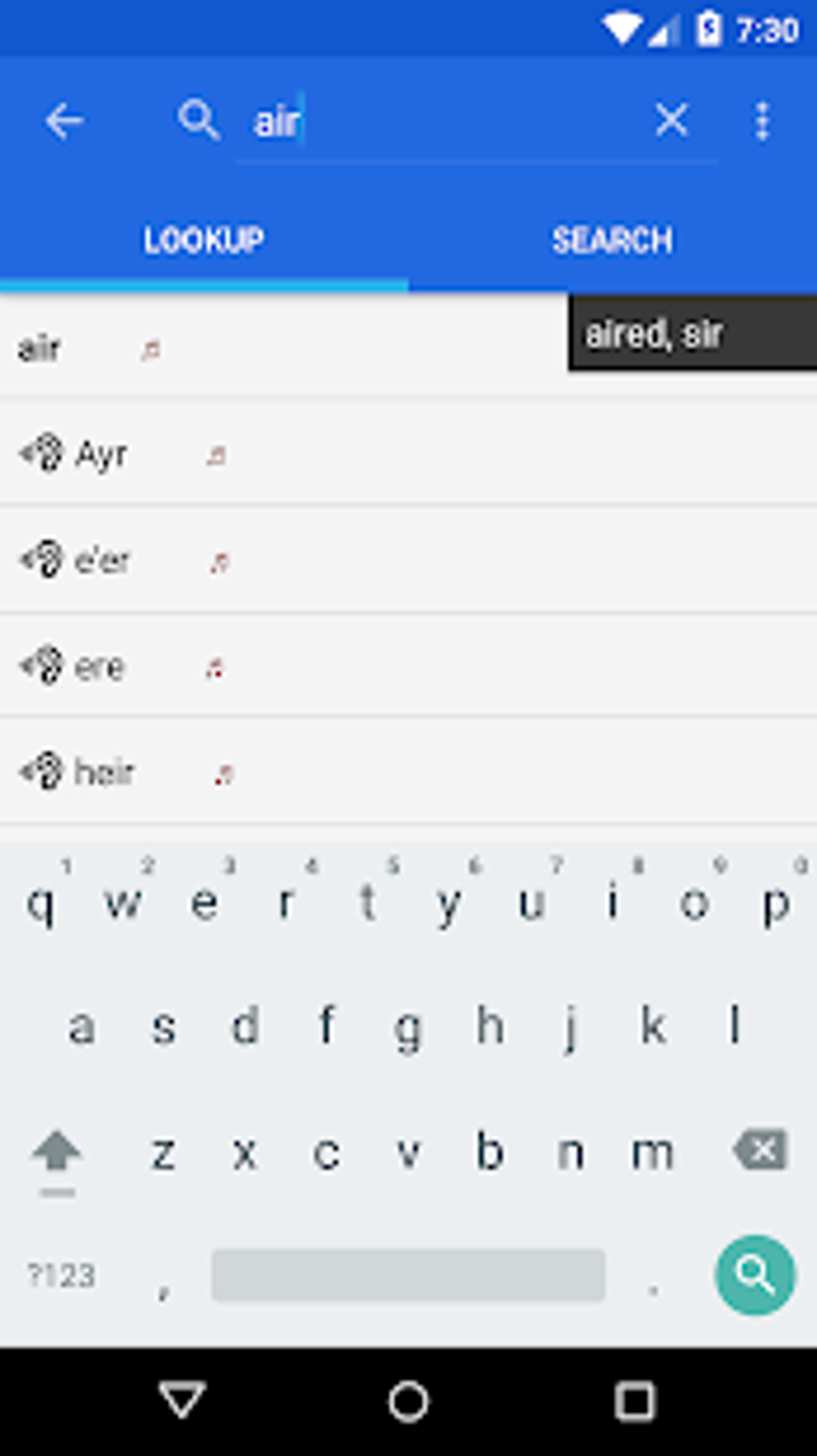A blurry and somewhat unclear screenshot taken from a mobile phone, displaying an application interface on the screen. At the very top of the screenshot, typical smartphone status icons are visible, including Wi-Fi connection, network connection, battery status, and the current time. The screenshot captures an application that appears to be a dictionary or word lookup tool, currently showing search results for the word "air" with different spellings and possibly different languages. The bottom portion of the screenshot reveals the digital keyboard, occupying the lower part of the screen, along with the standard navigation buttons for Android devices: an upside-down triangle, a circle, and a square. The overall color scheme of the screenshot is predominantly blue and grey.